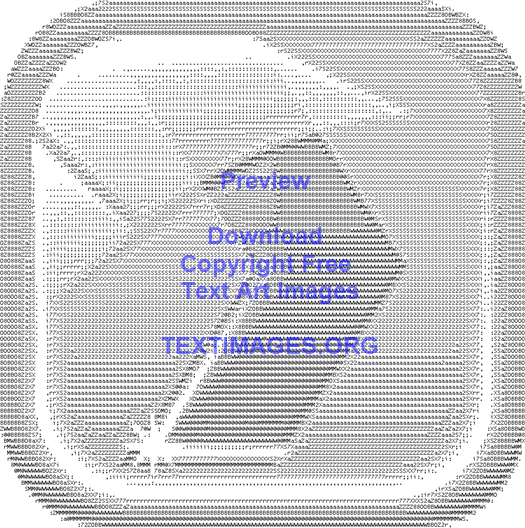This image features a logo-like design composed entirely of keyboard characters, forming a large square with a right-pointing arrow within it. The design is created using a pixel art style with a monochrome palette of black, white, gray, and bluish-purple. Dominating almost the entirety of the photo, this intricate text art piece also includes a centrally placed watermark that reads, "Preview, Download copyright-free text art images, textimages.org." The overall presentation suggests an advertisement for a website that offers text-based art images.